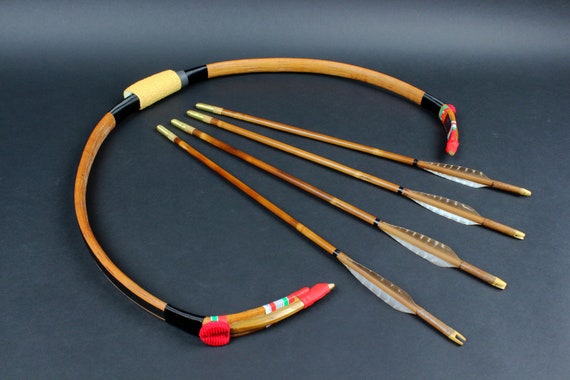The image displays a semi-circular wooden object resembling an incomplete bow, lacking the usual bowstring, adorned with red, white, and green decorative edges and a black-taped handle. Inside the open curve of the bow, there are four tan-colored darts or arrows, each with notched ends and small feathers in shades of brown and gray. The tips of these arrows are blunt. The background of the image is a dark gray gradient, which brightens towards the top, highlighting the objects.